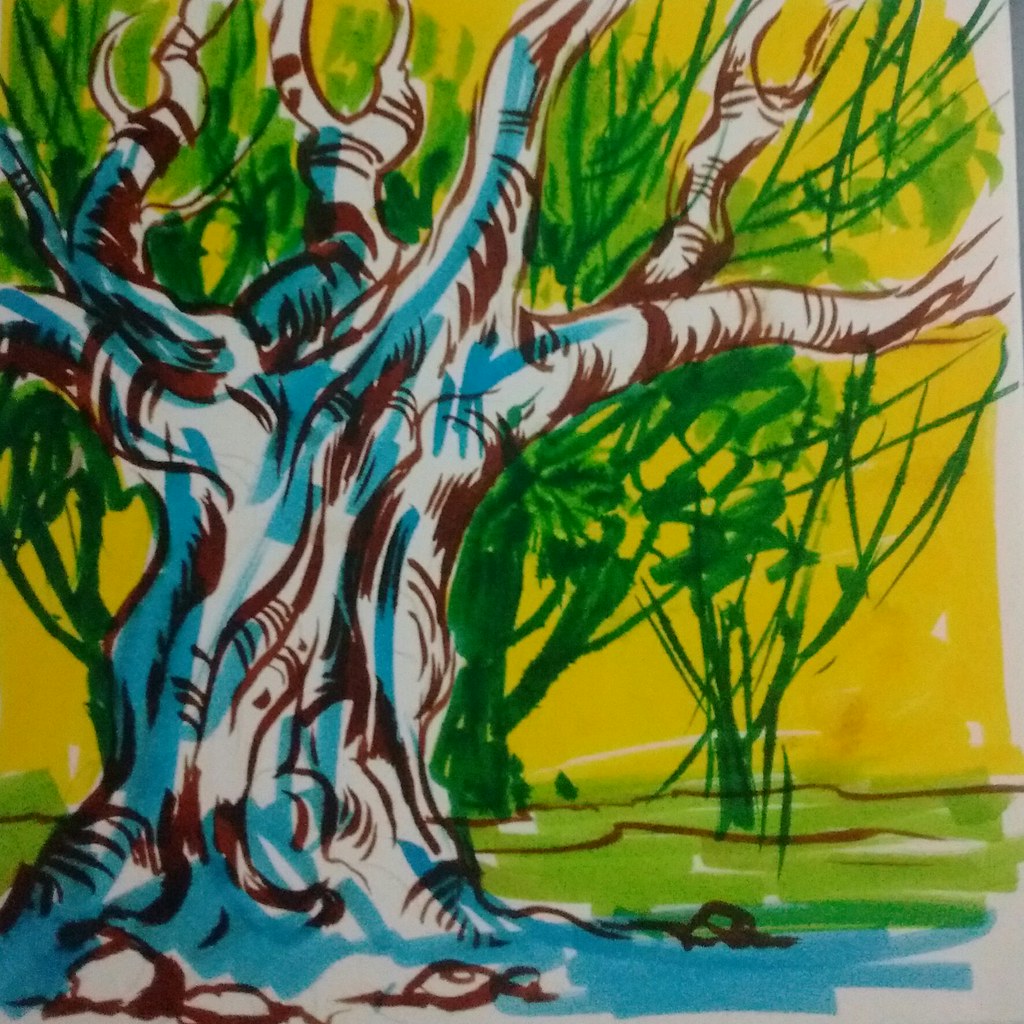This vibrant image depicts a large tree, artfully illustrated using what appears to be colorful magic markers. The solid hues suggest the use of ink rather than crayon. Dominantly, the tree showcases a blend of brown and white, skillfully shaded in blue, presumably from the same markers. Its base is sturdy, branching out haphazardly in all directions. Surrounding the branches, there are scribbles of green, possibly representing foliage from another tree in the background. Interestingly, this tree itself lacks any green leaves. The ground beneath it is illustrated in green, providing a sense of grounding to the artwork. The background is filled with a solid yellow color, adding a vibrant and lively dimension. On the right edge of the image, the white border of the paper is visible, giving a glimpse of the artist's canvas.